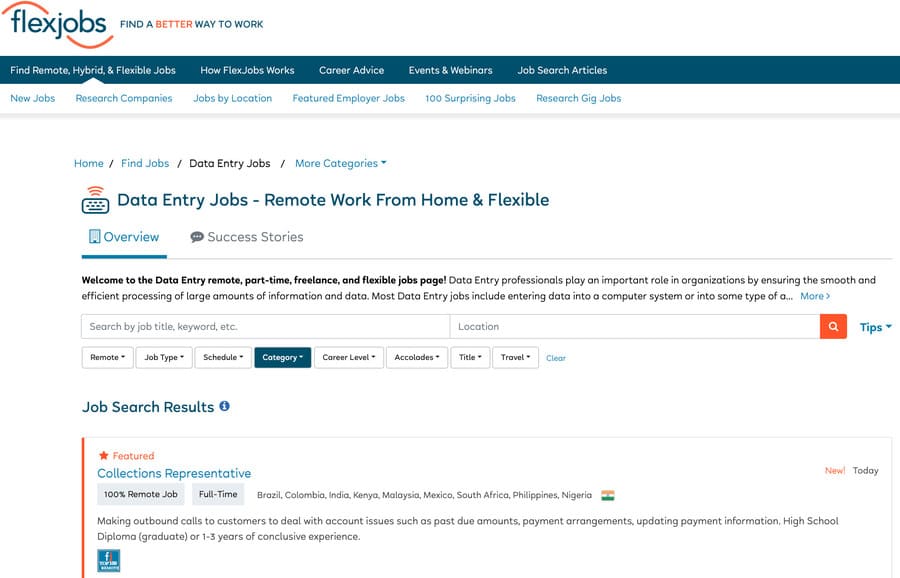This image is a detailed screenshot of the FlexJobs website homepage, meticulously designed and structured for user engagement. At the top, a distinctive logo featuring "Flex" in blue font with an orange semi-circular squiggle facing downward, and "Jobs" also in blue with the matching squiggle inverted, draws immediate attention. The tagline "Find a better way to work" is prominently displayed, with "better" highlighted in orange while the rest of the text is in blue.

A blue navigation banner at the top of the page provides quick access to various sections with white text: "Find Remote, Hybrid, and Flexible Jobs," "How FlexJobs Works," "Career Advice," "Events and Webinars," and "Job Search Articles." Below this, a white secondary banner categorizes more specific options such as "New Jobs," "Research Companies," "Jobs by Location," "Featured Employer Jobs," "100 Surprising Jobs," and "Research Geek Jobs."

The main content below these banners indicates that the user is on the "Data Entry Jobs" section, highlighted in black in a navigation menu while the rest of the categories, including "Home," "Find Jobs," and "More Categories," remain in blue. The header reads, "Welcome to the Data Entry Remote, Part-Time, Freelance, and Flexible Jobs Page," followed by an extensive introduction with an invitation to explore further by clicking "Read More."

Below this header, there are two long search bars for entering job titles, keywords, and locations, each extending across the page with an orange magnifying glass icon for initiating the search. Additional options for filtering jobs by various categories such as remote work type, job type, schedule, and career field are available, with selected categories being highlighted in blue.

At the bottom, the "Search for a Job" results appear under a white banner. The highlighted job, "Collections Representative," is marked with an orange star symbol to denote a featured listing, alongside descriptive text detailing the job location and specifics.